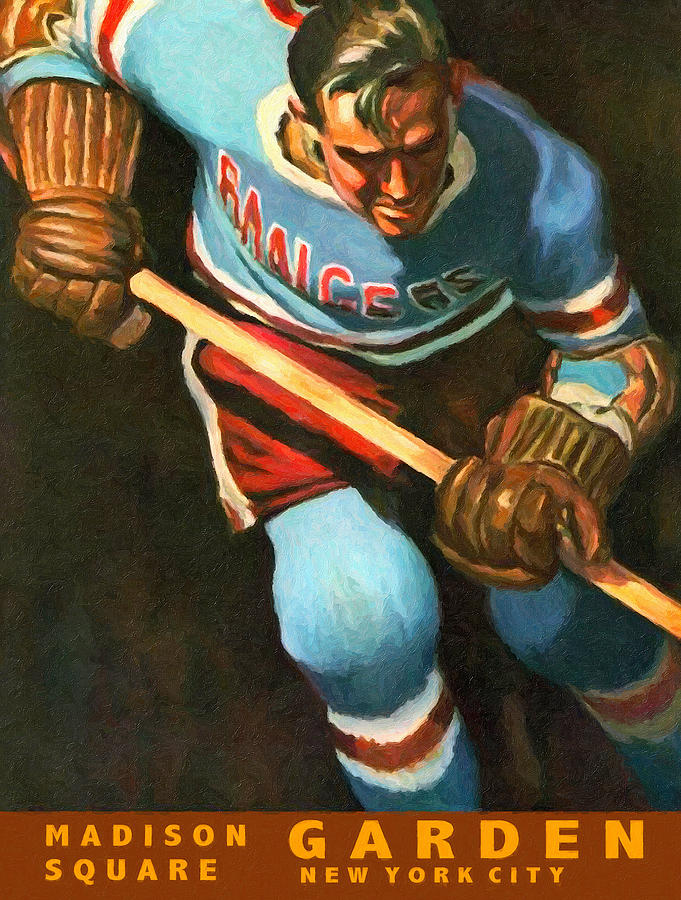This poster is a vintage-styled, oil-painted artwork for the New York Rangers hockey team, prominently displaying a scene at Madison Square Garden, New York City. The central figure is a determined male hockey player with short blondish hair, captured mid-action as he skates, possibly chasing or pushing a puck. He is clad in a classic Rangers uniform featuring a baby blue jersey with red and white trim and stripes, red shorts, and blue pants adorned with white-red-white stripes at the bottom. The player also sports large, thick brown gloves. The entire scene is rendered in a palette that includes baby blue, brown, red, white, dark brown, and dark yellow. Notable is the bold, yellow text at the bottom of the poster, set against a brownish-orange background, reading "Madison Square Garden, New York City." The dynamic and vintage aesthetic of the artwork emphasizes the historical and spirited nature of the event.